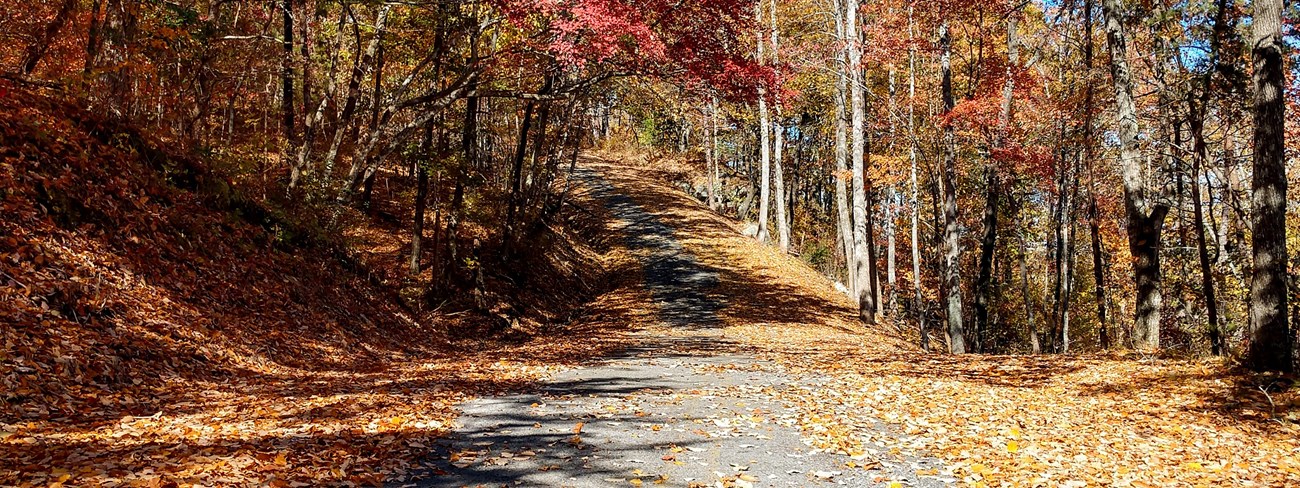This is an outdoor photograph capturing a picturesque autumn scene in a wooded area. The wide-aspect image showcases a country road or paved trail, covered in bright auburn, brown, red, yellow, and gold leaves, indicating the height of fall foliage. The road, a light gray tarmac, winds up a gentle hill before curving to the left, with shadows cast across its leafy surface. To the left of the road, there is a steep embankment densely populated with trees; vibrant red, muted yellow-orange, and olive green leaves adorn these trees, some of which are bare. On the right side, the landscape drops off into a downward incline, creating a contrast with the upward hill on the left. The sky is a clear blue, peeking through the canopy of trees and enhancing the rich autumnal colors that dominate the scene.